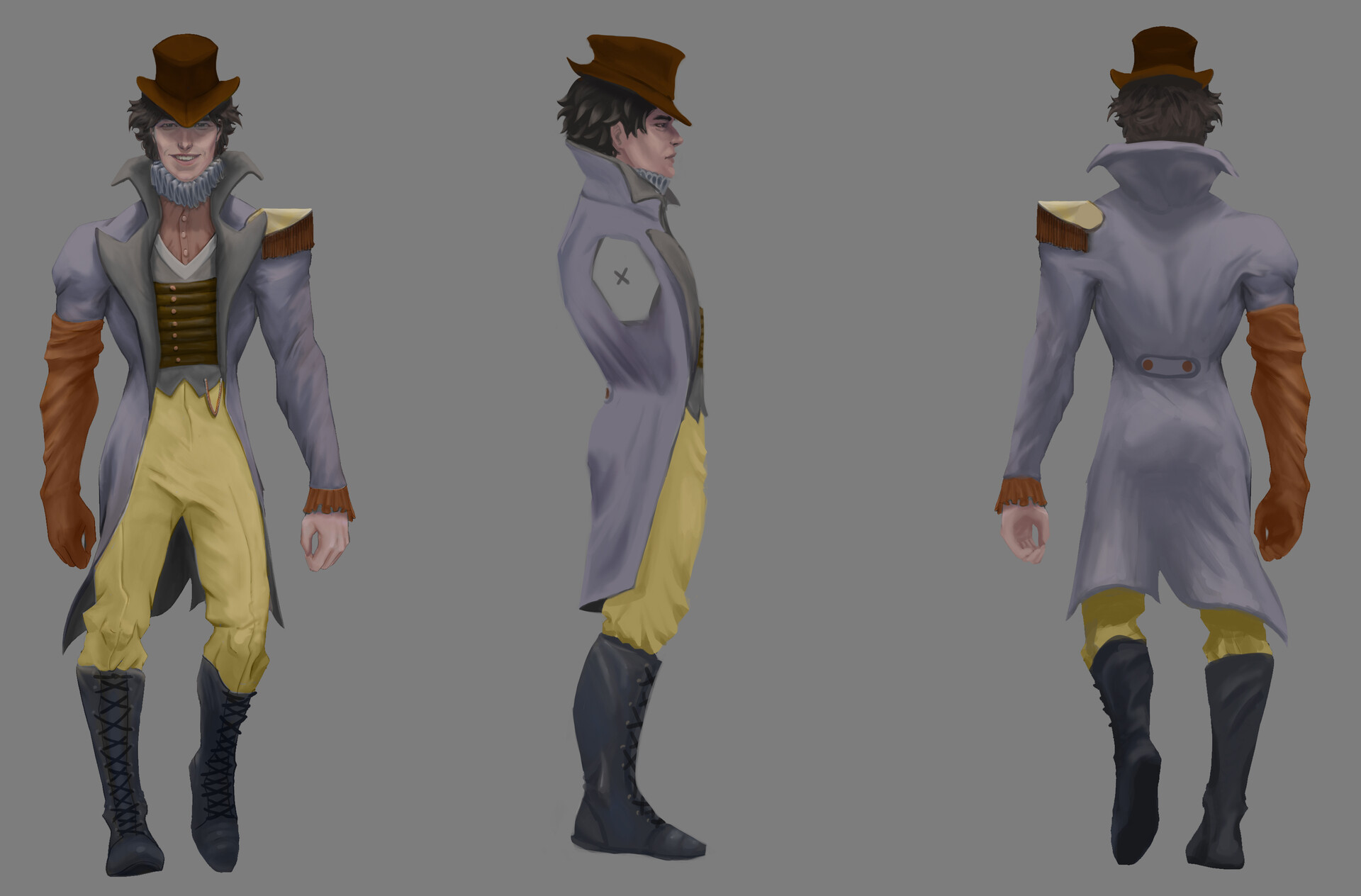This digital artwork depicts a man in three different positions: front, side, and back. The man is adorned in a distinct and eclectic outfit. Starting from the top, he wears a light brown top hat that reveals darker brown hair at the sides. A gray high-collared jacket with wide lapels drapes his upper body, and on the left shoulder, there's a prominent yellow square patch, while the purple sleeve on the right side adds an asymmetrical touch. Underneath the coat, a brown cummerbund extends over a gray vest and forms a V-neck pattern on his chest, accented by a dark decorative design. His neck is wrapped in a thick piece of material, enhancing his unique style.

Below, he sports form-fitting yellow pants tucked into blue boots. On his arms, there is a contrast: the right arm is covered with a long brown glove extending from the bicep to the fingers, whereas his left arm remains bare, except in the center pose where his left arm is replaced by a gray patch with a black X in place of his shoulder. 

From the back, the coat extends down to behind his knees, maintaining the high collar that wraps around his neck. Both his arms hang down by his sides, revealing the contrasting glove on the right arm and the bare left hand with peach-colored skin. His overall attire and the detailed differences in his poses capture the eclectic and somewhat whimsical nature of his fashion, reminiscent of late 1800s European style.